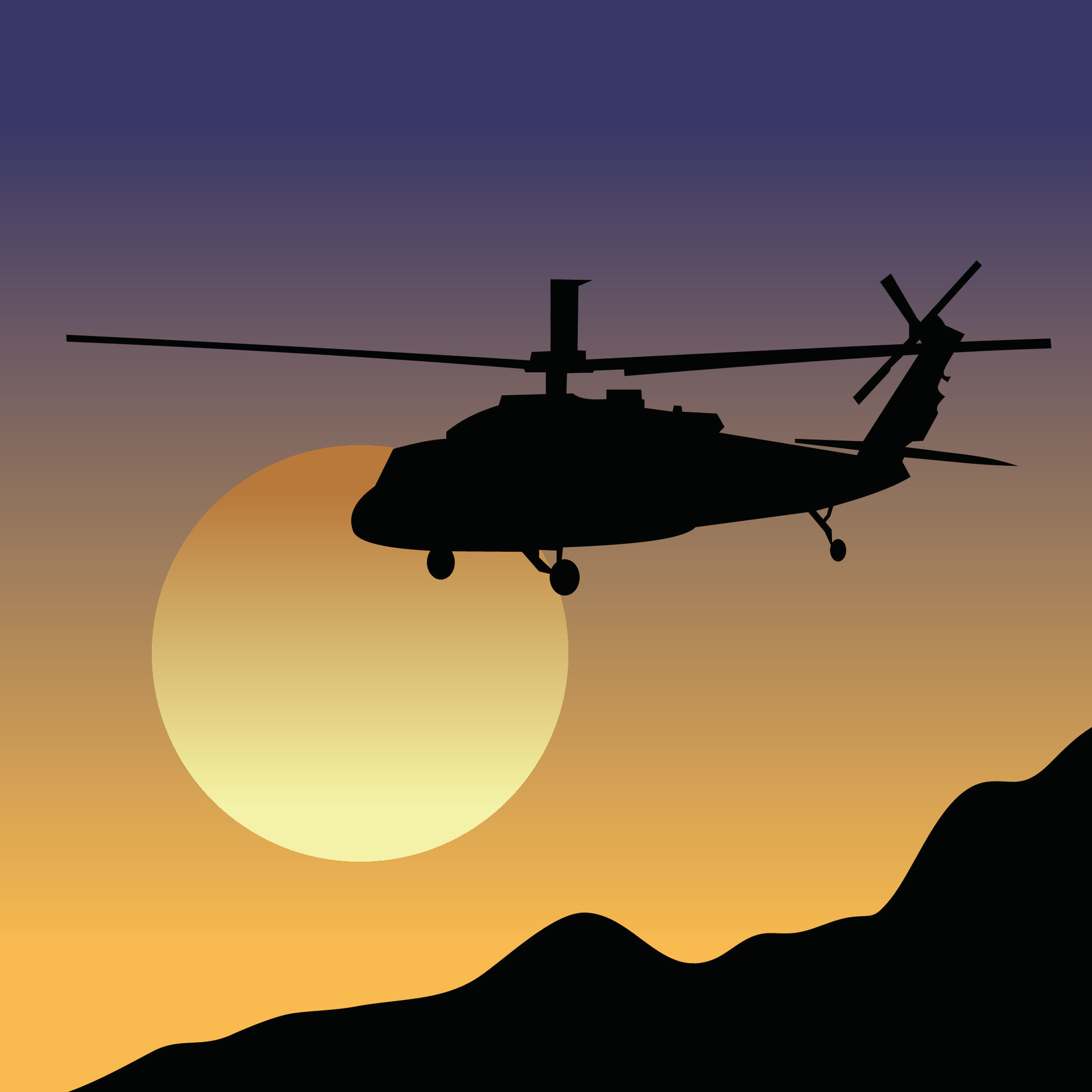This image depicts a stylized, computerized drawing of what appears to be an Apache-style military helicopter flying in front of a large, orange sun. The helicopter, rendered entirely in solid black, showcases a distinct outline without any interior detail, capturing its iconic silhouette with the prominent rotor blades. Its solid black form matches the silhouetted ridge line of mountains at the bottom of the image, adding a cohesive unity to the composition. The sky features a dramatic gradient, transitioning from a vibrant orange near the horizon to a deep purple at the top, conveying the atmosphere of a sunset or early evening. The vivid color gradient and simplified forms give the image a contemporary, almost poster-like appearance, emphasizing the stark contrast between the silhouetted figures and the richly colored sky.